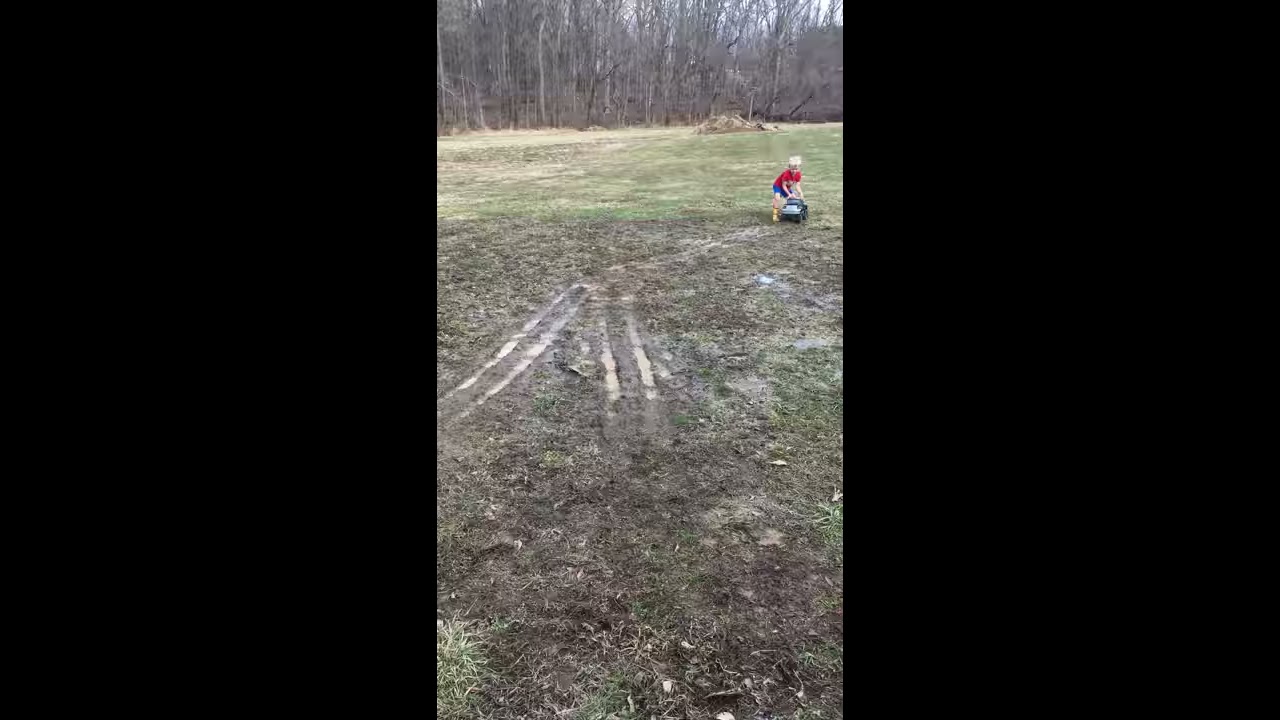In this photograph taken in the midst of the day, we see a young boy playing outdoors in what appears to be a muddy field, possibly his backyard. The field's surface is a mix of grass and mud, suggesting recent rain. The center of the image is dominated by a muddy patch with visible tire marks, likely made by the toy car the boy is pushing around. The boy, who is blonde and seems to be having fun, is positioned towards the top right of the image. He is wearing a red shirt, blue shorts, and yellow boots, and is holding a sizeable toy car. The background is filled with gray, leafless trees and bushes, with some sky poking through, indicating an overcast or early spring setting. The scene is devoid of text, showcasing a natural palette of colors including black, brown, green, tan, red, blue, yellow, and gray.